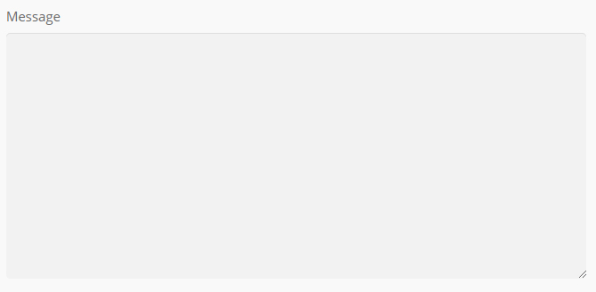The image depicts a rectangular text box with the word "Message" located at the top-right corner of the box. The text box itself is slightly gray, standing out against its off-white background. The off-white border surrounding the text box is relatively thin on all sides except for the top, which is designed significantly larger to accommodate the word "Message" in gray font. Notably, the text box appears to be empty and includes a small corner with two subtle diagonal lines, suggesting a design element or a placeholder. It seems as though this text box has been clipped from a different webpage, highlighting its horizontal orientation as the longer side, compared to the shorter vertical side.